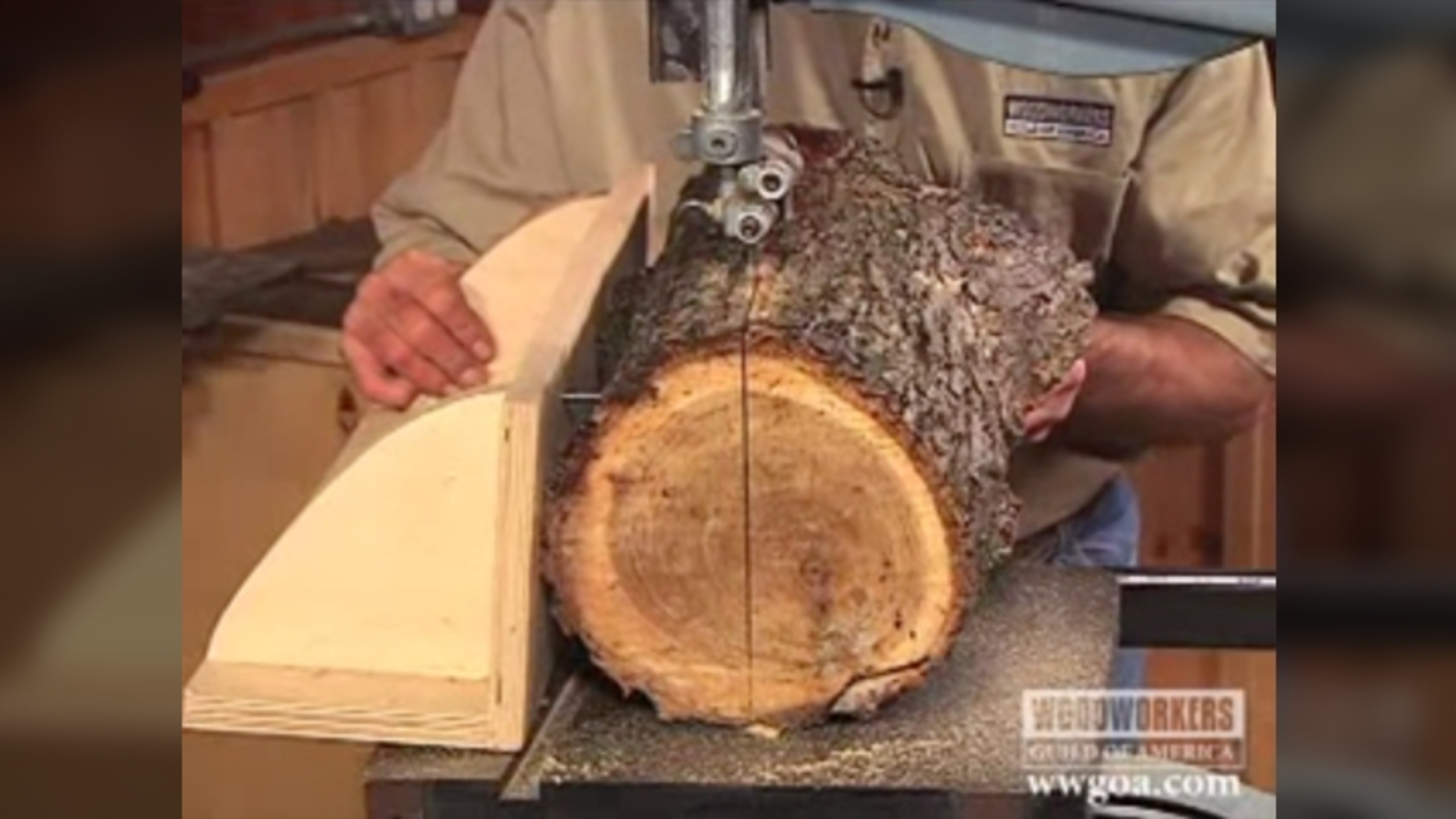The image depicts a person engaged in woodworking, specifically cutting a thick log in half using a large bandsaw. The individual is wearing a tan t-shirt with a label on the top left side, though the head and face are not visible as they are cut off from the frame. The picture has a blurry quality overall, with the left and right sides particularly more out of focus, creating a somewhat fragmented appearance. The center of the image, while still slightly blurry, shows the person standing behind the bandsaw, guiding the log through the cut. The log retains its bark and measures approximately a foot in width. In the bottom right corner, there is a watermark featuring the text "Woodworkers Group of America" in white, followed by the URL "www.goa.com."